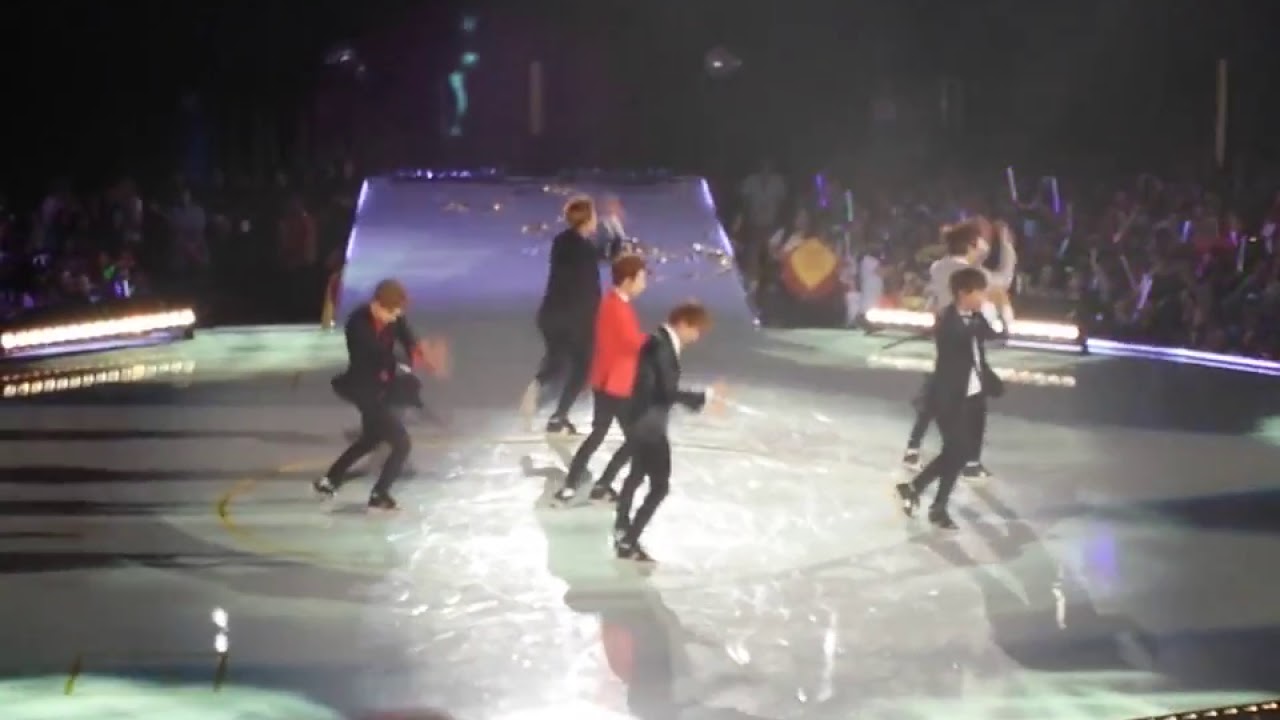The image depicts a dynamic stage performance taking place in an indoor setting. The rectangular photograph, approximately six by four inches, focuses on a circular stage viewed from a side angle. The stage is crowded with young men, seemingly of Asian descent, arranged in a structured formation. The main stage area is circular until it extends upwards into a ramp at the center, leading off to the left. 

On the stage, there are six performers dressed in formal attire, suggesting a dance or possible tap dance routine. They are positioned in three staggered rows: one man in the back left row, three men in the middle row slightly left of center, and two men in the front row to the right. Most are wearing black or dark gray suits with the exception of one man in a red jacket situated at the center of the middle row, and another man in the front row rightmost position who contrasts with a light, possibly stone-colored jacket. One particularly enthusiastic performer on the leftmost side is notably more bent and energetic in his movements, clapping vigorously.

Surrounding the stage is a crowded audience, with attendees holding vibrant light sticks, predominantly in pink and purple hues, particularly concentrated on the right side. The top left section of the stage's ramp features a person dressed in a glowing green outfit, adding a distinct splash of color. The backdrop suggests that the performance is well-received, as the audience appears highly engaged, emphasizing the impressive and lively atmosphere of the event.